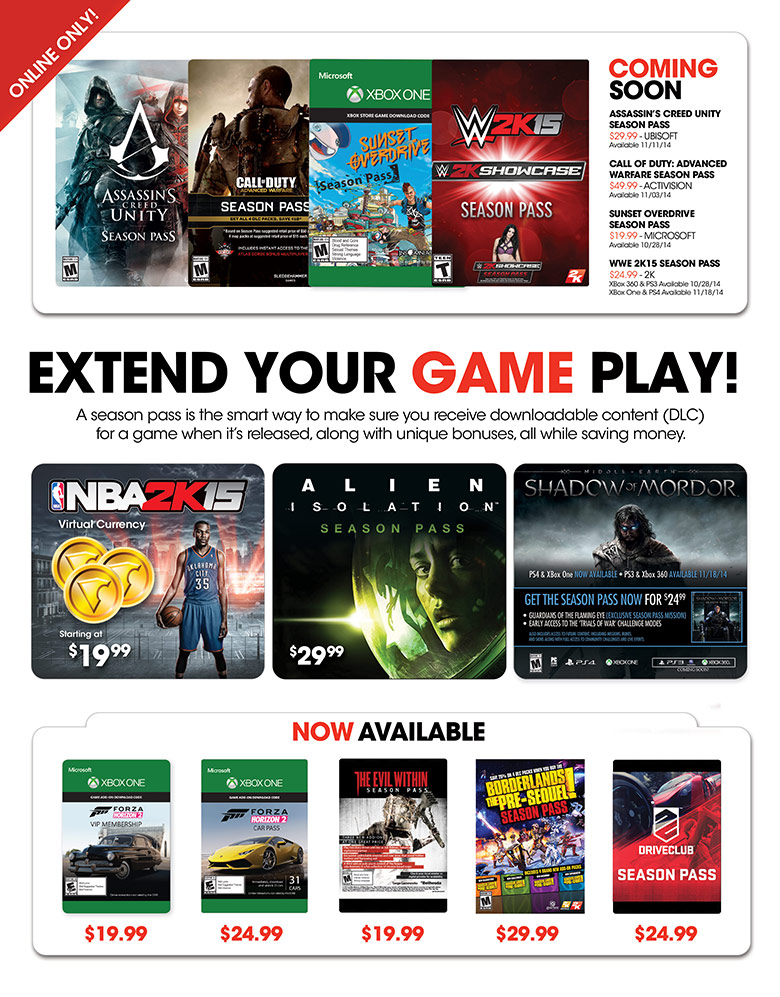In this promotional poster, prominently displayed in the top left corner is the phrase "Online Only." The poster highlights various video games that come with season passes, offering extended gameplay through downloadable content (DLC). Featured games include "Assassin's Creed Unity" with its Season Pass, "Call of Duty: Advanced Warfare" with its Season Pass, and "Sunset Overdrive" for the Microsoft Xbox One, also available with a Season Pass. Further, games like "WWE 2K15" (represented as W2K15) come with a "W2K Showcase" and a Season Pass. 

The poster emphasizes the benefits of purchasing a Season Pass, stating that it ensures access to all upcoming DLC and exclusive bonuses, ultimately saving money. Also shown are "NBA 2K15," "Alien Isolation" with its Season Pass, "Shadow of Mordor" for Xbox One, as well as "Forza Horizon 2," which includes a Car Pass and VIP Membership. Moreover, "The Evil Within" is listed with its Season Pass, "Borderlands: The Pre-Sequel" with its Season Pass, and "Driveclub" also with a Season Pass. Pricing details for these offers are mentioned at the bottom of the poster.